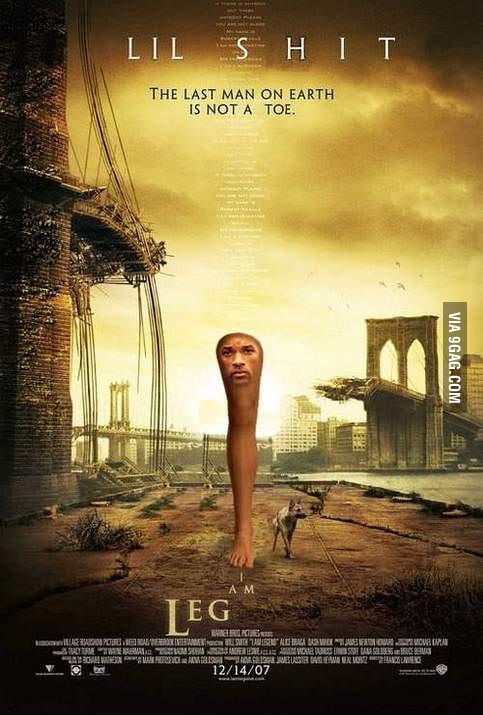The image is a parody movie poster of "I Am Legend", titled "I Am Leg" with the release date 12-14-07. The poster features a sepia-toned, apocalyptic background with a cloudy sky, depicting a partially destroyed city in the distance and a broken bridge. In the foreground, there is a peculiar and humorous twist: instead of Will Smith, it showcases a single leg with Will Smith’s face positioned at the knee. Next to the leg stands a black dog, reminiscent of the movie's iconic canine companion. The top of the poster reads "LIL SHIT" in large capitals, followed by the subcaption "The last man on earth is not a toe." Various colors are visible, including shades of brown, yellow, orange, white, black, and gray. This playful and surreal image mimics the original "I Am Legend" promotional material but with an absurd, comedic alteration.